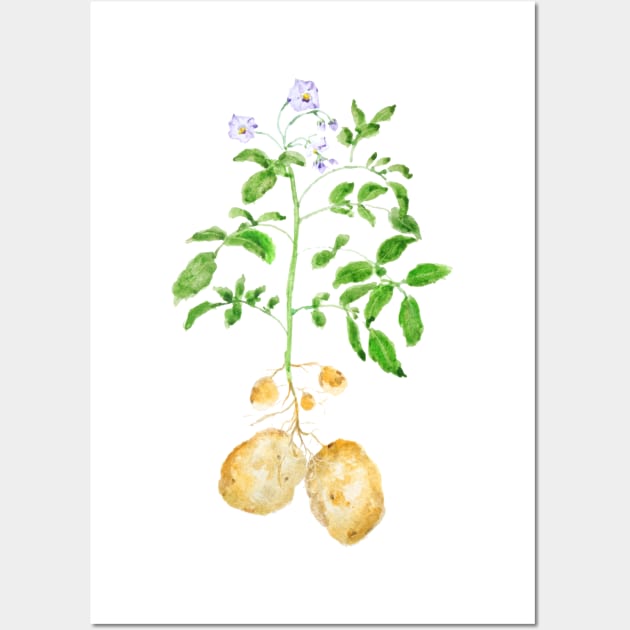The image showcases a painting or drawing on a rectangular, white canvas displayed against a white wall with light gray vertical strips on either side. The artwork features a detailed potato plant emerging from the bottom, with several large brown potatoes attached to its roots. The plant's green shoots and small green leaves spread out in various directions. At the top of the plant, there are about 5 to 6 flowers, painted in hues of purple with yellow centers; two of these flowers are fully bloomed, while the others are still budding. The canvas itself stands out due to its even brighter white hue in contrast to the white wall behind it.